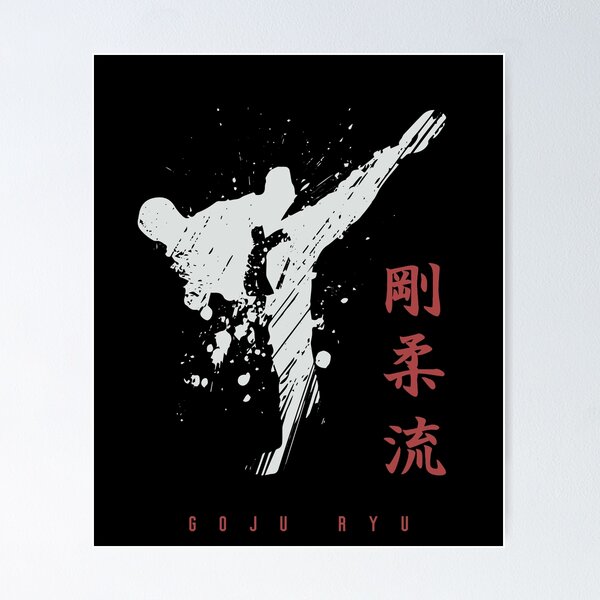This image features a dynamic promotional poster for a martial arts studio or event, with a stark black background accentuating the central figure. The white-painted, impressionistic silhouette depicts a martial artist in a gi, adorned with a black belt, performing an impressive high kick with their left leg extended well above their head. Scattered splashes of white paint artfully define the figure's form, adding an abstract allure to the image. Adjacent to the martial artist, three vertical red kanji characters enhance the poster with an authentic touch, possibly indicating the martial art's name or philosophy. At the bottom, also in red, the text "Goju Ryu" is prominently displayed, suggesting a connection to this particular Karate style. The vivid contrast and minimalistic design elements make this poster a striking and effective visual representation of martial arts prowess and discipline.